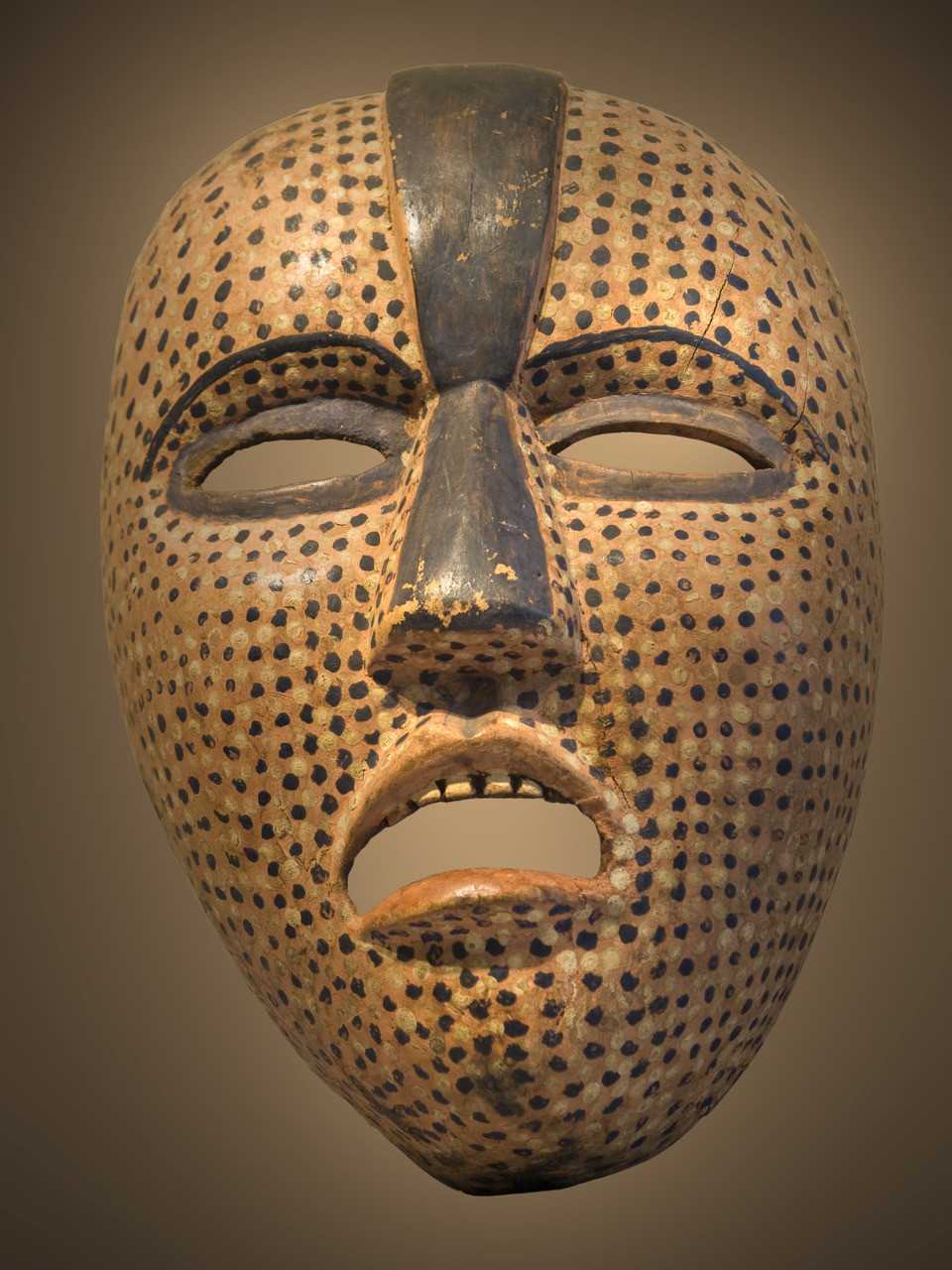This photograph depicts an ancient tribal mask, likely of African origin, exhibiting clear signs of wear and weathering that suggest its age. The mask, which appears to be carved from wood, is predominantly light brown or beige with an intricate pattern of variously colored dots across its surface. These dots are mostly black and dark brown interspersed with yellow, white, and lighter beige dots. A prominent black or dark brown stripe runs from the top of the forehead down to the tip of the nose, which includes a slight protrusion. The eyes are bordered with the same dark color, while thin, curved eyebrows are painted above in dark brown. The mask has a partially open mouth revealing four upper teeth, contributing to its somewhat stern or angry expression. The backdrop for this mask is a grayish-brown wall, mostly shrouded in shadow, adding depth to the overall appearance. The craftsmanship and detailed decorations suggest this mask could be a museum-worthy artifact.